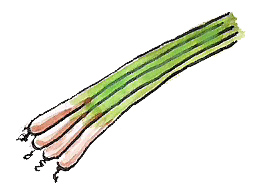This image is an illustration of four spring onions, also known as green onions or scallions. The drawing features four distinct stalks, each outlined in black, with the white bulbs positioned towards the bottom left corner. The bulbs have small, fine roots depicted in a fuzzy black texture. About a third of the way up the stalks, the white bulbs transition into long green stems, which angle upward towards the top right. The green areas are vivid and clear, although the overall style maintains a charming, cutesy feel. The shadows of the white bulbs are accented with a brownish-red hue, suggesting depth. The illustration is set against a plain white background, with no additional elements, and while the exact medium is unclear, it appears reminiscent of watercolors.